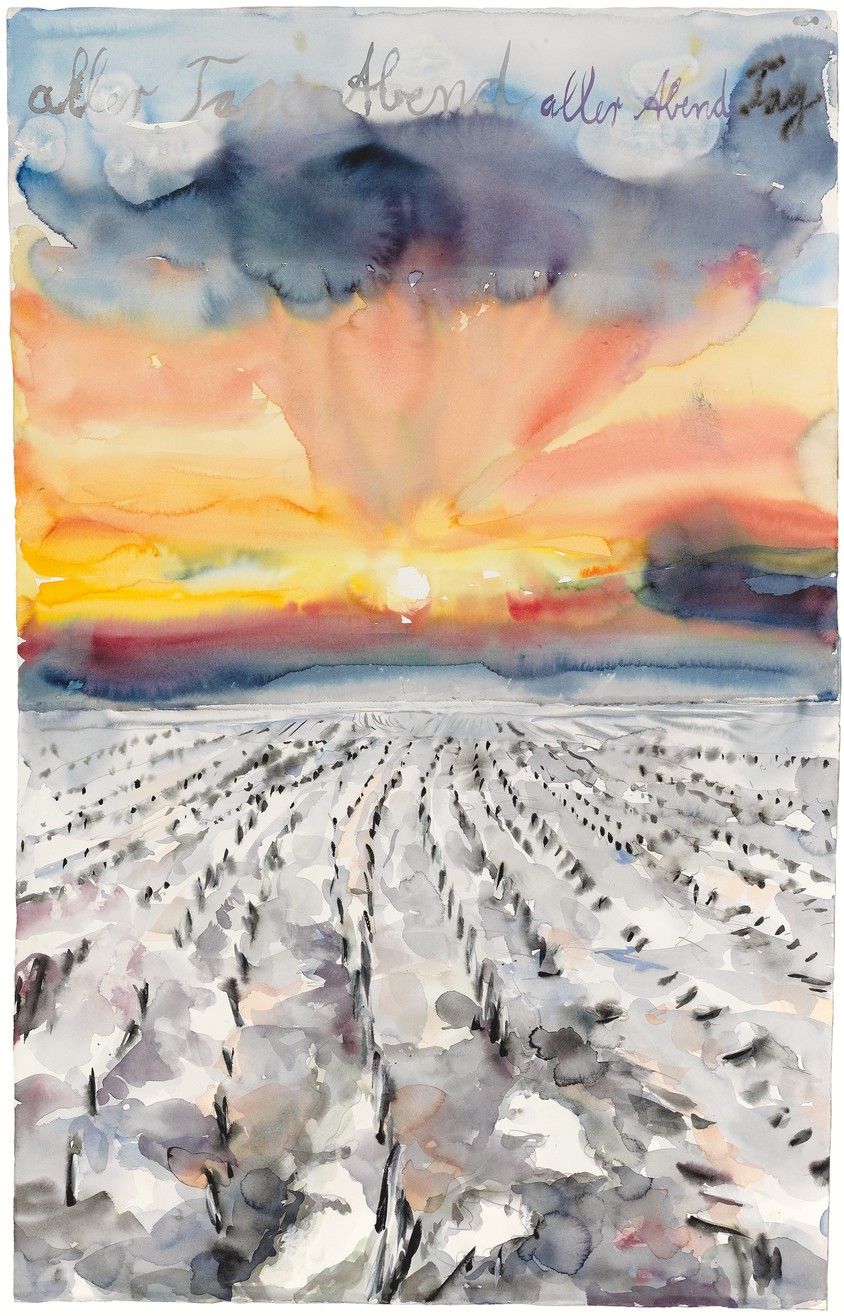This intriguing image presents an impressionistic, watercolor landscape titled "The Evening of All Days, The Day of All Evenings." The bottom half of the image depicts a snow-covered farm field with rows of harvested stumps or branches emerging from the pristine white blanket of snow. In the mid-section, the horizon is defined by dark hills, subtly lit by the sun, which is either rising or setting. The light from the sun floods the scene in a spectrum of vibrant colors, ranging from bright orange and yellow near the horizon to shades of pink and midnight blue as it ascends. A dazzling display of orange splashes against the hills, creating a dynamic contrast with the serene snow-covered field below. The sky is a captivating gradient, starting from the brilliant oranges near the sun and transitioning to darker hues and whites at the top, interspersed with clouds tinged with gray and silver. Above this intricate palette, some German cursive writing adds a final touch of mystery and sophistication to the artwork. The combined elements of the farm field, vibrant sunset, and evocative use of colors create a vivid and harmonious visual experience.